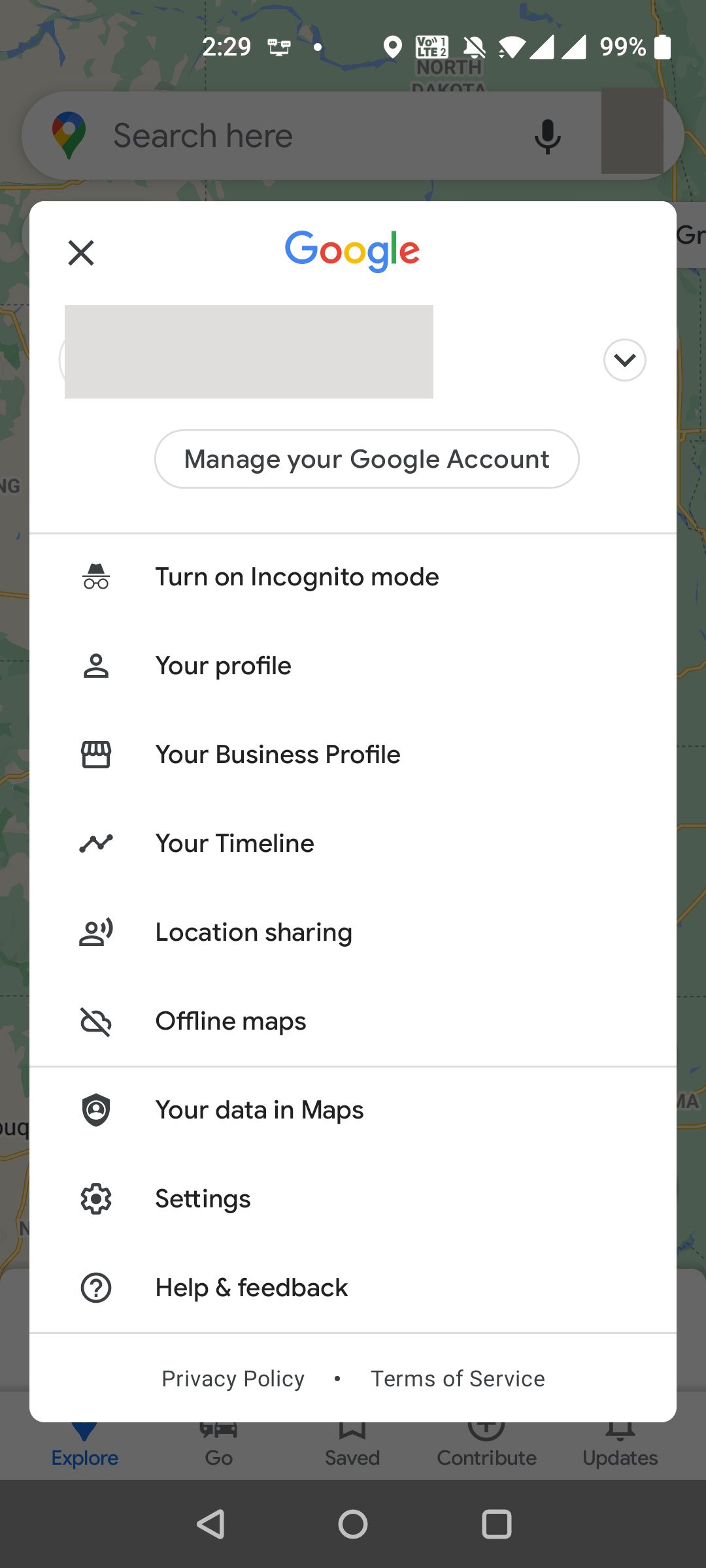A screenshot of a smartphone displays the Google Maps application prominently. At the top, a notification indicates a voicemail is waiting, while a small icon shows that notifications are silenced. The device is connected to Wi-Fi and the battery is fully charged at 99%.

The background features a detailed map with a distinct Google Maps pin. The map view is partially obscured by a Google pop-up window, marked with an 'X' in the corner for closing. The pop-up includes the iconic Google logo in its trademark colors: blue, red, yellow, green, and again blue, green, and red.

Below the logo, a gray search bar invites users to explore. A drop-down menu offers a range of options: Manage Your Account, Turn on Incognito Mode, Your Profile, Your Business Profile, Your Timeline, Location Sharing, Offline Maps, Your Data in Maps, Settings, and Help and Feedback. At the bottom of the menu, links to the Privacy Policy and Terms of Service are visible.